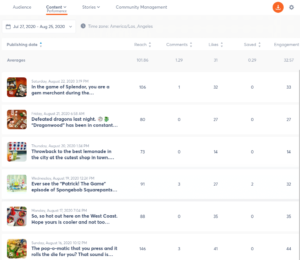This is a detailed caption:

"A screenshot of a web page with extremely small and blurry text, making it difficult to read. In the upper left corner, there are four tabs labeled 'Audience,' 'Content' (with a dropdown menu and a word underlined with an orange line beneath it), 'Stores,' and 'Community Management.' An orange, circular button with a downward-pointing arrow is present in the top left area. The content of the web page is indecipherable, but it appears to be related to recipes or possibly instruction manuals for home craft projects."